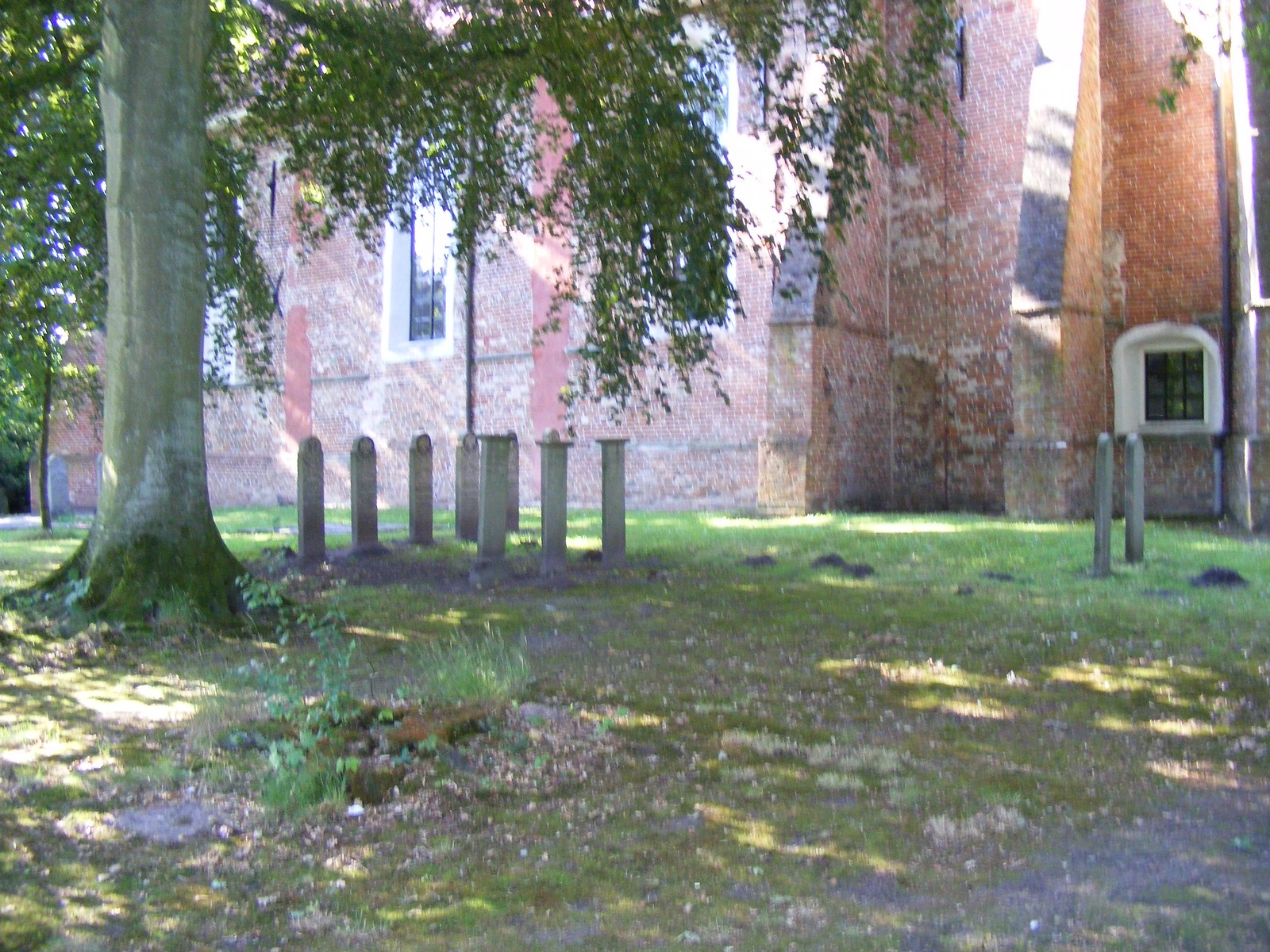This horizontal, color photograph captures an outdoor scene dominated by a large, red brick building with weather-beaten bricks that suggest its age. The building features several long, narrow windows with white moldings and black grids that divide the panes into small squares. In front of the building, there is a grassy area interspersed with patches of dirt, stones, and weeds. Prominent in the foreground is a large tree on the left-hand side, with its trunk extending upwards and branches with green leaves reaching across the top and left edges of the frame. Surrounding the tree and scattered throughout the grassy space are several vertical, slate-gray objects that appear to be oblong stones with possible engravings, which could be gravestones, implying the area may be a cemetery. A notable concentration of these stones is visible to the right and back of the tree, with a few additional stones closer to the right-hand side of the photograph.